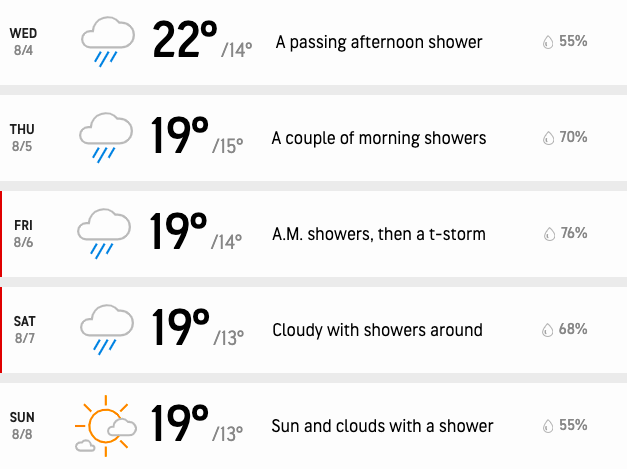This image displays a detailed five-day weather forecast for a specific region, presented against a white background with black and grey font. 

Starting from the left, the forecast for Wednesday, August 4th, shows an icon of a cloud with blue rain lines, indicating a passing afternoon shower. The temperature is forecasted at a high of 22°C and a low of 14°C, with a 55% chance of precipitation, represented by a raindrop symbol.

Moving to the right, Thursday, August 5th features a cloud with rain lines, predicting a couple of morning showers. The temperatures will range from a high of 19°C to a low of 15°C, with a 70% chance of rain.

Next, Friday, August 6th, marked by a red line, continues the trend with another cloud and rain icon. The temperature is set to be 19°C during the day and 14°C at night. The forecast notes morning showers with a possible thunderstorm, with a 76% chance of precipitation.

On Saturday, August 7th, the weather remains cloudy with rain, as shown by the cloud and rain icon. The high will be 19°C and the low 13°C. The description says "cloudy with showers around," and the chance of rain is 68%.

Finally, Sunday, August 8th displays a mix of sun and clouds with a small chance of a shower. The icon shows a sun with rays peeking through clouds. The temperatures will be 19°C for the high and 13°C for the low, with a 55% chance of rain.

This structured and detailed forecast helps in planning for the week, with varying chances of rain and temperatures staying fairly consistent.